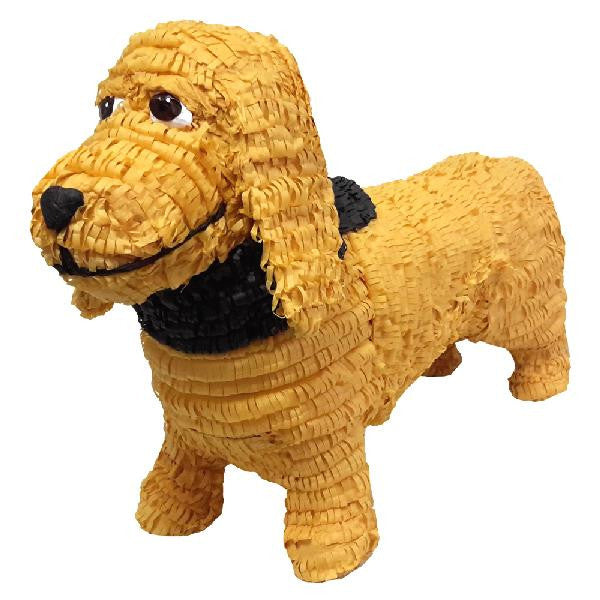The image features a detailed pinata in the shape of a dachshund, showcasing golden, retriever-like fur made from papery, tissue material commonly used in pinatas. The dog, characterized by its elongated, wiener dog body and one prominently visible floppy ear, gazes towards the left. Its eyes, boasting white backgrounds with either brown or black irises, appear quite expressive. The pinata sports a black bandana or scarf wrapped around its neck, with the same color extending underneath and partially on the back of the neck, giving it a small and endearing look. The dog’s face is neutral, with a subtle smile and a black nose, enhancing its lifelike yet cartoonish appearance. The background is stark white, drawing full attention to the intricately designed pinata with its short, curly fur texture.